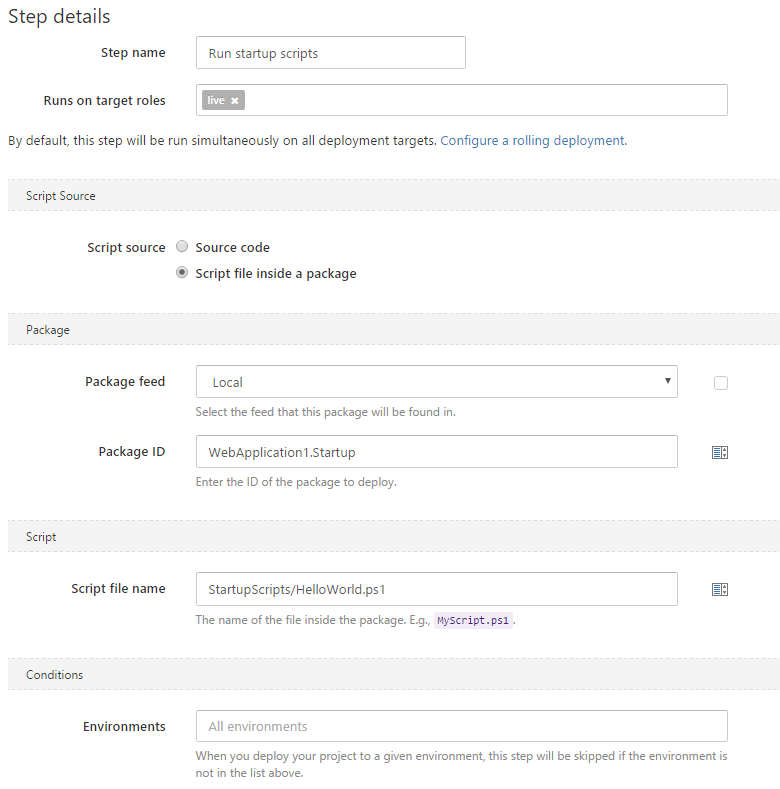This image is a detailed screenshot of a form interface with a white background and bluish-gray text. The upper left corner displays the title "Step Details." Below this title is a form section. The first line of the form reads "Step Name," and within its input box, the text "Run Startup Scripts" is entered. Below this, the label "Runs on Target Roles" appears, with a corresponding form box that contains a small gray box labeled "Live."

Underneath this form section, there is an informational message that states, "By default, this step will run simultaneously on all deployment targets," followed by a link in blue text that says "Configure a Rolling Deployment."

Further down, a light gray banner contains the text "Script Source." Beneath this banner, the form segment labeled "Script Source" offers two options: "Source Code" and "Script File Inside a Package," with the latter being blacked out, indicating it is currently selected or inactive.

Lastly, another gray banner labeled "Package" is present. Below it, the "Package Feed" section features a dropdown box that displays the word "Local" along with a pull-down arrow, indicating more options are available.